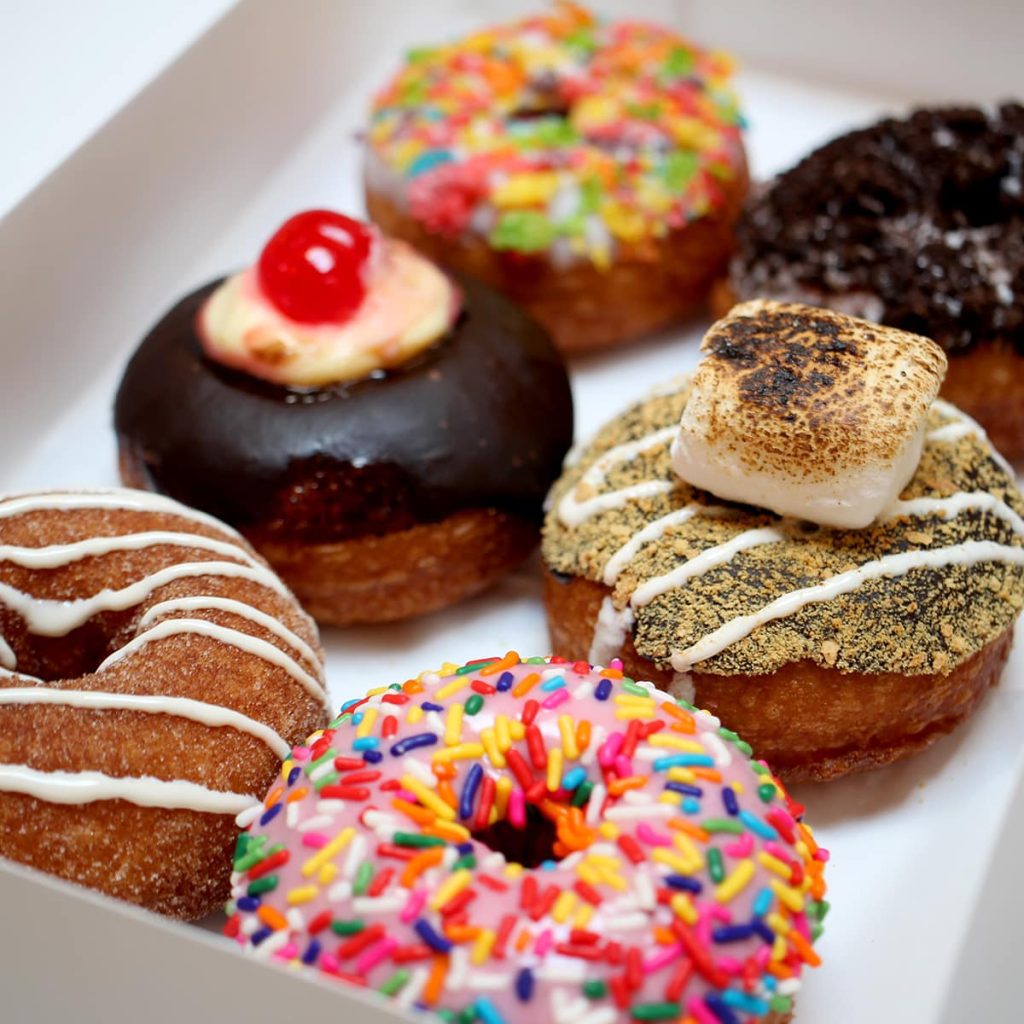This vibrant and detailed photograph captures an assortment of six distinct donuts arranged in a slightly askew white box, with the length of the box pointing towards the upper right. The focus is centered on the middle donuts, while those at the edges blur slightly. In the top left corner, a donut with a rainbow array of red, yellow, green, blue, pink, and purple sprinkles stands out. To its immediate right, a donut sits adorned with white frosting and dark chocolate sprinkles. The middle left donut is a decadent creation with a base of chocolate frosting, topped with a dollop of white cream and crowned with a maraschino cherry. Sliding to the middle right, the donut features a dark chocolate glaze, light brown dusting, white frosting drizzled artistically, and a toasted marshmallow perched on top, evoking a s'mores theme. In the lower left, a brown sugar donut is drizzled with white frosting, providing a simple yet appealing look. Finally, the bottom right donut bursts with color, covered in pink frosting and topped with multicolored sprinkles featuring shades of red, orange, yellow, green, purple, and light blue. Each donut not only contrasts in flavors and decorations but also contributes to the overall vibrancy and depth of the image.